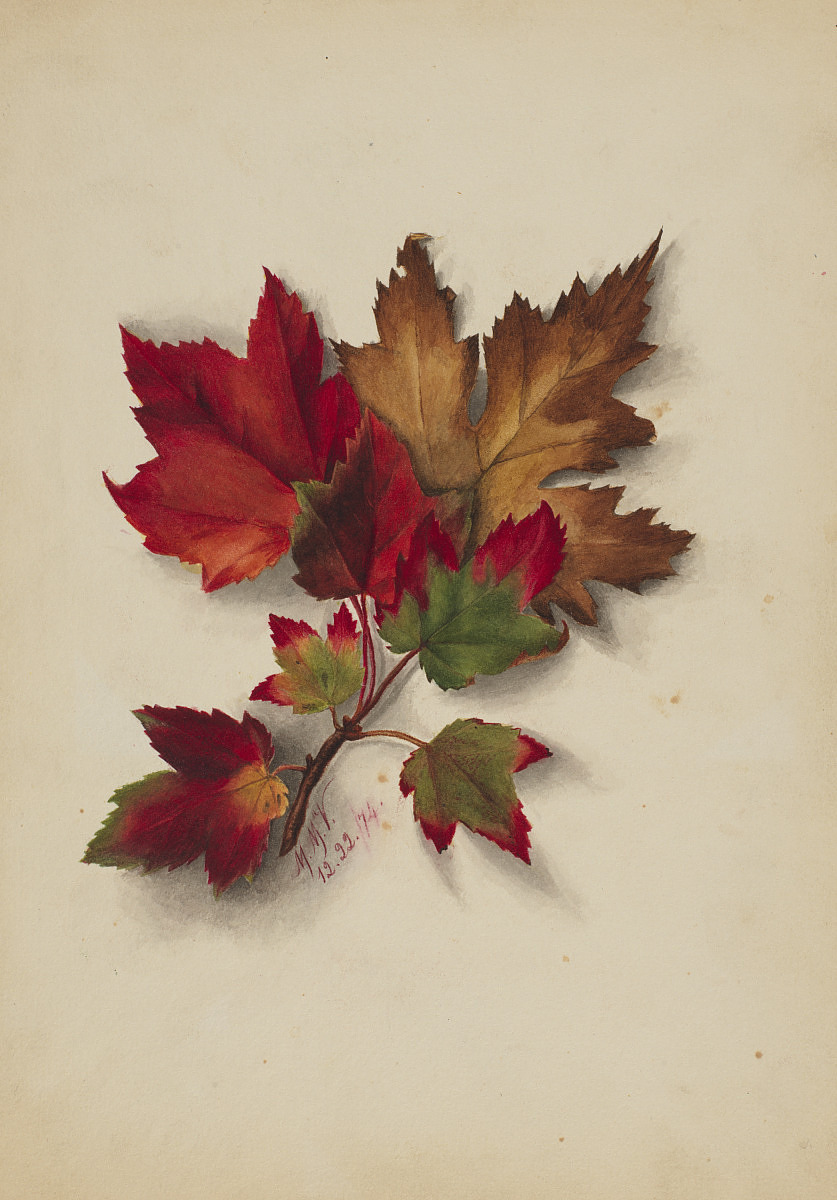The image is a vertically rectangular painting set against a plain, dark cream background. It features a single twig adorned with several autumn-colored leaves, positioned centrally and pointing diagonally toward the top right corner. The entire twig is about three inches long. At the bottom left of the twig, there's a red leaf with a green tip, while just above it sits a smaller green leaf with red tips. Directly to the right of these leaves is another green leaf with red tips, and slightly above it, a larger green leaf with red tips can be seen. Toward the middle left, there is a red leaf with one green tip, and above it, another red leaf, slightly larger, overlaps with a smaller red leaf. The top of the twig is crowned with a prominently large brown leaf, suggestive of decay. The leaves feature a range of colors including green, red, yellow, and brown, typical of the fall season. In the bottom right corner of the painting, a signature reads "MMV 122274," indicating the artist and date, December 22, 1974.